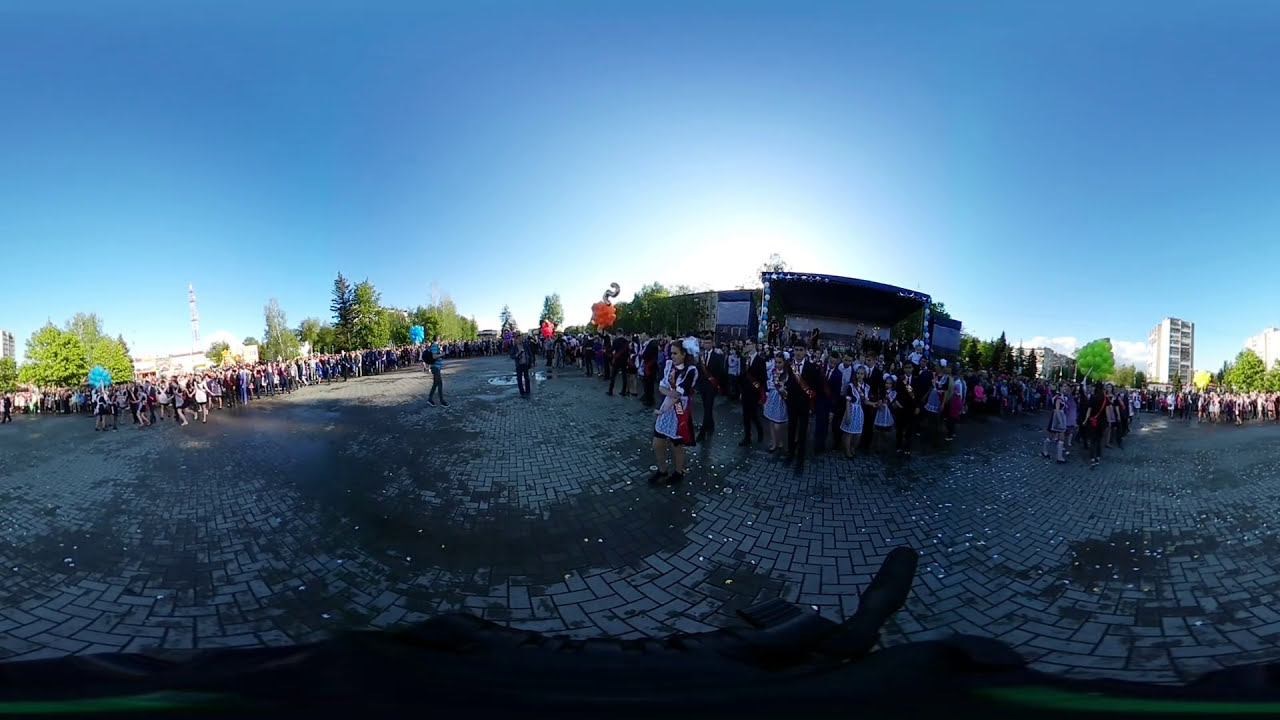The photo captures a large outdoor gathering on a wet brown cobblestone surface with sporadic pieces of paper or trash scattered across it. The image is taken at an angle, placing most of the numerous attendees—estimated to be in the hundreds—in shadow, despite the bright, clear blue sky overhead. The crowd, consisting mainly of men in black tuxedos and women in black dresses with white, ruffled aprons resembling maid outfits, stretches broadly across the scene. They're gathered around a dark, square building with distinctive orange and red accents, as well as blue markers dotted nearby. Surrounding the area are green trees, and in the distance to the far right, a tall building is visible. Additionally, another building with a tower is partially seen on the far left, framing the scene as a busy, expectant crowd stands amidst well-illuminated natural surroundings.